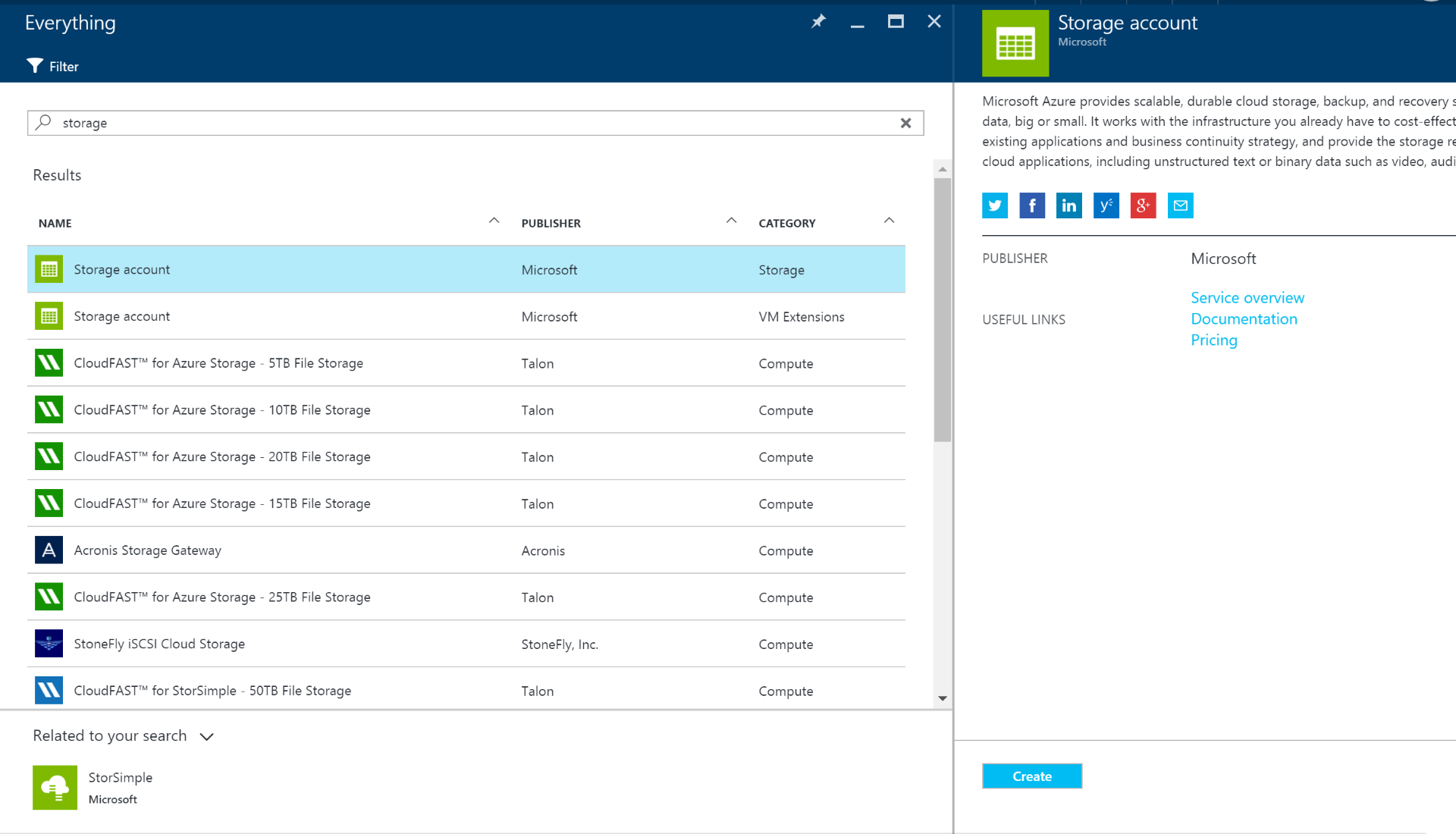This screenshot is of a website interface primarily focused on storage management. In the top left corner, the website's title, "Everything," is displayed, potentially indicating comprehensive storage search functionality or a storage software named "Everything." Just beneath this title is a filter button, suggesting options to refine search results.

Directly below the filter button is a search bar with the term "storage" entered, hinting that the user is searching for storage-related items. The search results show a highlighted entry labeled "Storage Account," distinguished by a light blue hue indicating the current selection or hover state.

The entries underneath "Storage Account" include another category titled "VM Extensions." Each listing is organized with headers such as "Name" on the left, "Publisher" in the center, and "Category" on the right. Among these listings, there's a repetitive entry type labeled "Cloud Fast for Azure Storage," appearing multiple times with identical publishers and categories. The repeated entries differ only in storage capacity, suggesting they represent various terabyte options.

Overall, the website seems to be a cloud storage management or search tool, offering users the ability to filter and navigate through different storage options.